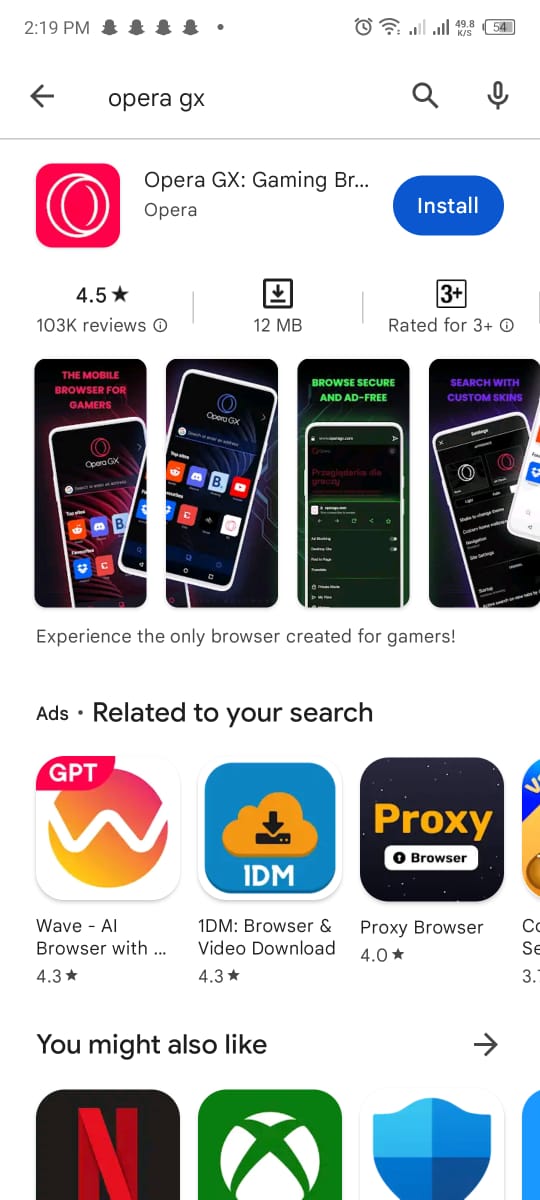The image is a screenshot of an application store on a mobile phone, showcasing the Opera GX browser. At the top of the screen, there is a white header with a gray arrow pointing left, followed by gray text that reads "Opera GX". To its right, there is a gray magnifying glass icon and a gray microphone icon. Beneath this header is a thin gray line.

Below the header, detailed information about the Opera GX application is displayed. On the left, there is a reddish-pink square with rounded corners featuring a white, angled doughnut-shaped logo. To the right of this logo, the app's title, "Opera GX: GamingBrew...", is written in gray text, with "Opera" in lighter gray text beneath it. To the right of these texts is a blue "Install" button with white text.

Further below is a section divided into three columns of information. The left column shows a rating of 4.5 stars with 103k reviews, accompanied by an eye icon encircled by a gray doughnut. The middle column, separated by a thin vertical gray line, displays a dark gray box with a downward arrow and a horizontal gray line, indicating the app's size of 12 megabytes. The right column, again separated by a vertical gray line, features a gray box with a "3+" symbol, signifying that the app is rated for users aged 3 and above.

Underneath this triptych of information, there are four images, each slightly separated by a white background. These images contain various photographs and labels, with the leftmost image having red text, the next with no text, the third with green text, and the rightmost image with purple text. 

At the very bottom of the screen, in light gray text atop the white background, there is the tagline, "Experience the only browser created for gamers."